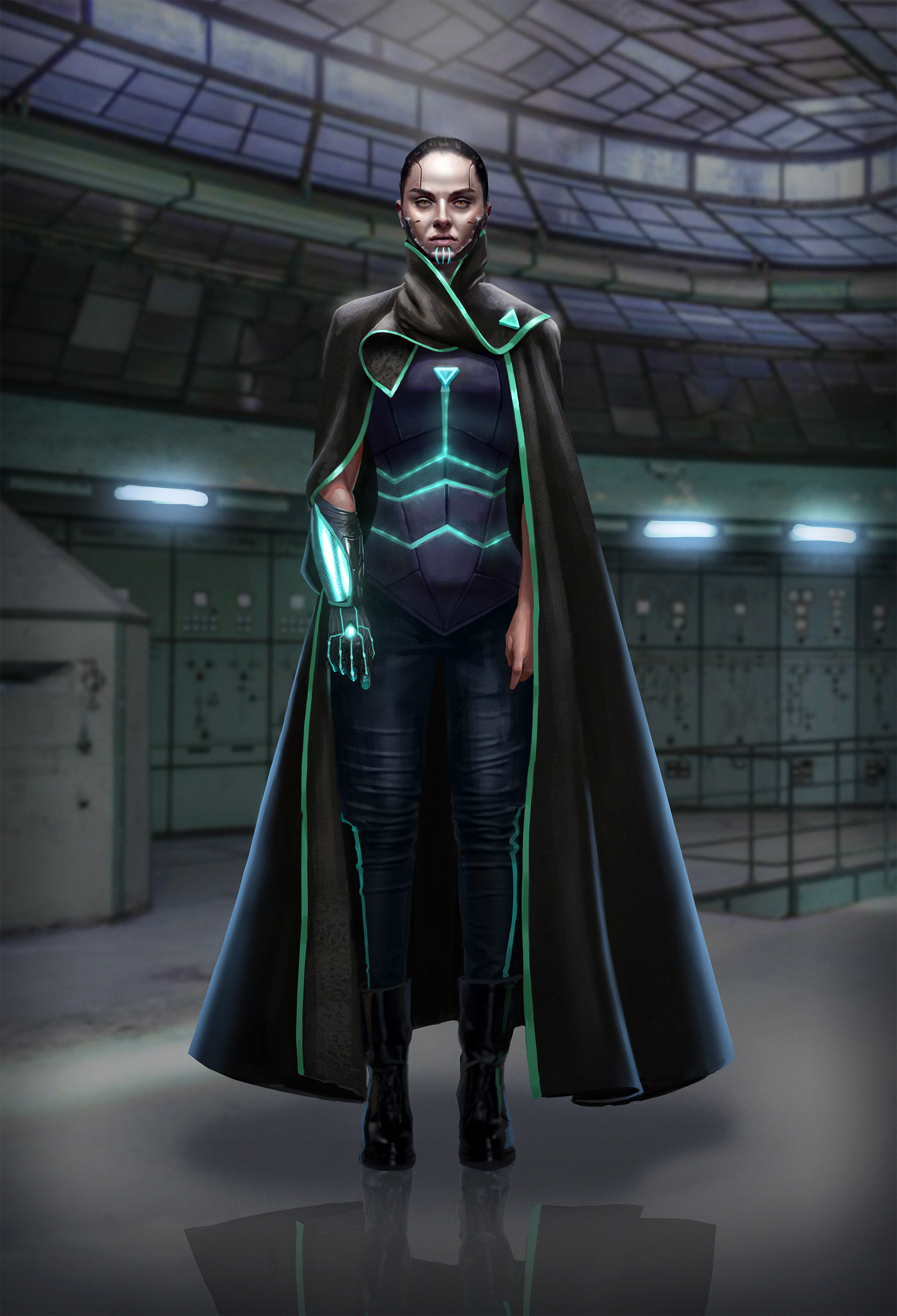The image appears to be an AI-generated depiction of a character from a sci-fi video game. The figure, who has androgynous features but leans towards a feminine appearance, stands facing the viewer in a futuristic setting that resembles a bunker or spaceship. She is dressed in an all-black tight suit akin to a wetsuit, adorned with green stitching, and wears a matching black cloak with green trim. Her right arm, from the elbow to the fingertips, is clearly robotic and features illuminated green accents, suggesting cyberkinetic enhancements. Her left hand, also robotic and gloved, peeks out from the cloak. She has her hair slicked back, enhancing her intense, focused gaze. The background is a machine-filled room with neon lights and intricate design elements, including a reflective linoleum floor and a domed glass ceiling composed of numerous panels intersected by black lines.